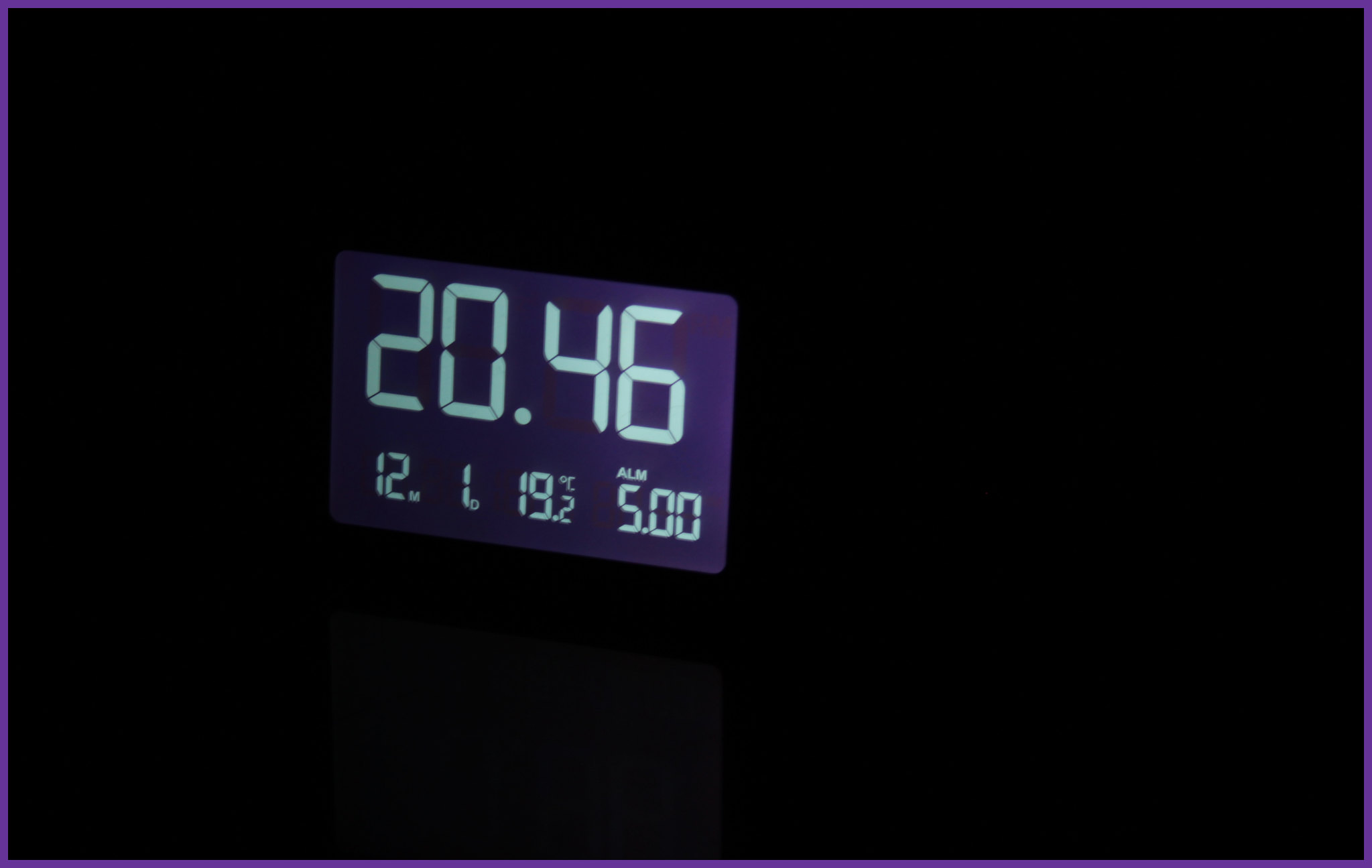This image portrays a distinctive digital alarm clock against a completely black background, suggesting it might be a digital creation rather than a conventional photograph. The edges of the screen are framed with a bright purple border, enhancing the modern aesthetic. The central display of the alarm clock has a dark purple hue. The time is prominently shown as 20:46 in a mix of white and teal digits, indicating military time. Additional information is displayed in smaller text at the bottom and right of the screen, including "19.2°C" for temperature and "ALM 5:00" indicating an alarm set for 5:00 a.m. A faint reflection is visible beneath the screen, adding a subtle hint of realism to the otherwise digital appearance. The image focuses solely on the screen and slight reflection, omitting any other part of the alarm clock.